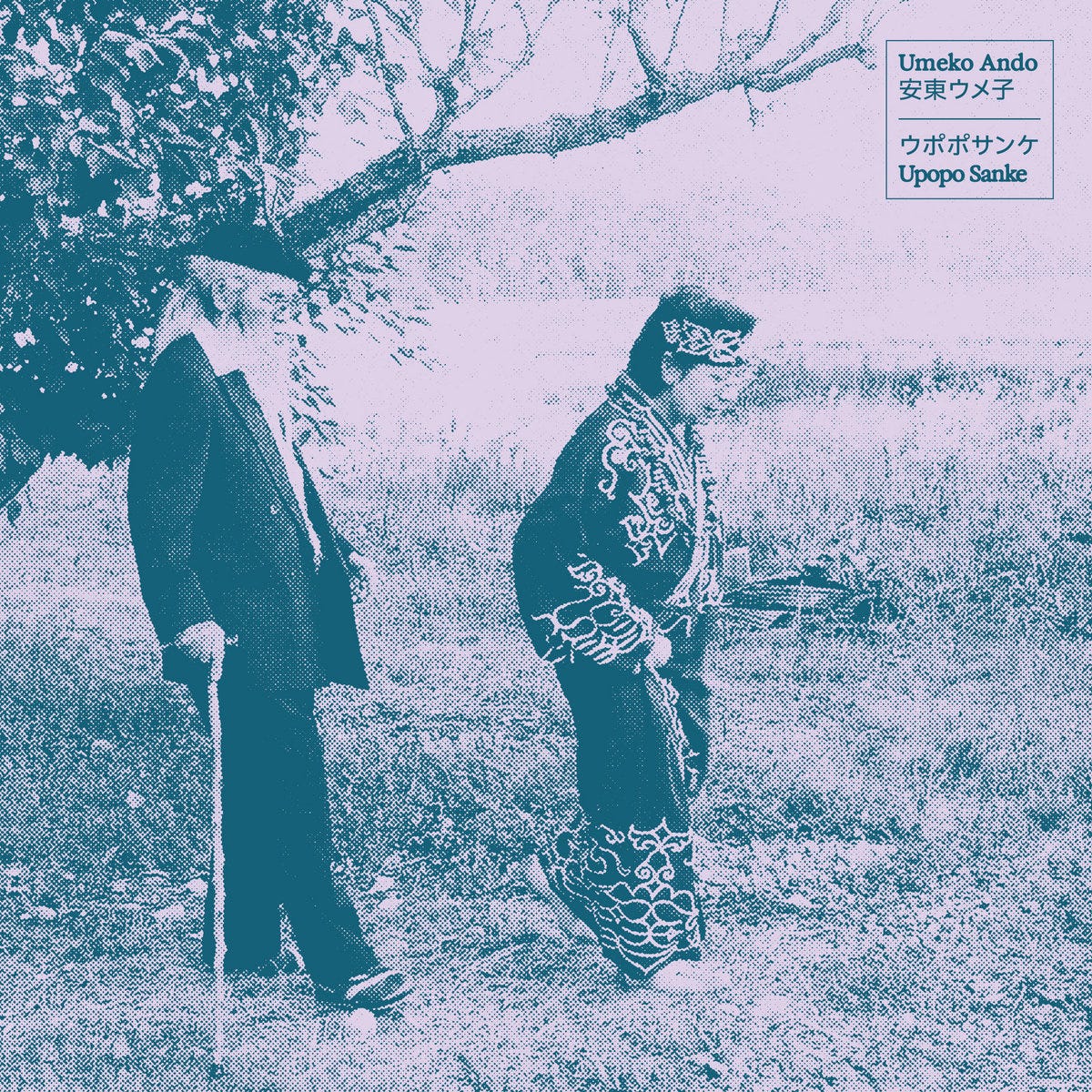This aged, black-and-white photograph, likely taken in Japan, is grainy and faded. At the top right, a square box contains the names "Yumiko Ando" and "Upopo Sanki," alongside Japanese characters. The image captures an elderly man and a woman walking in a grassy field under a tree with a large, bare branch extending to the right. The man, positioned to the left and slightly behind the woman, wears a black suit, a black hat, and glasses; he has a long white beard and hair and leans on a cane. The woman, in front, is adorned in a dark-colored kimono with intricate light-patterned embroidery and appears to be barefoot, although it's difficult to discern completely. Both individuals exude an air of traditional elegance juxtaposed against the serene natural backdrop.